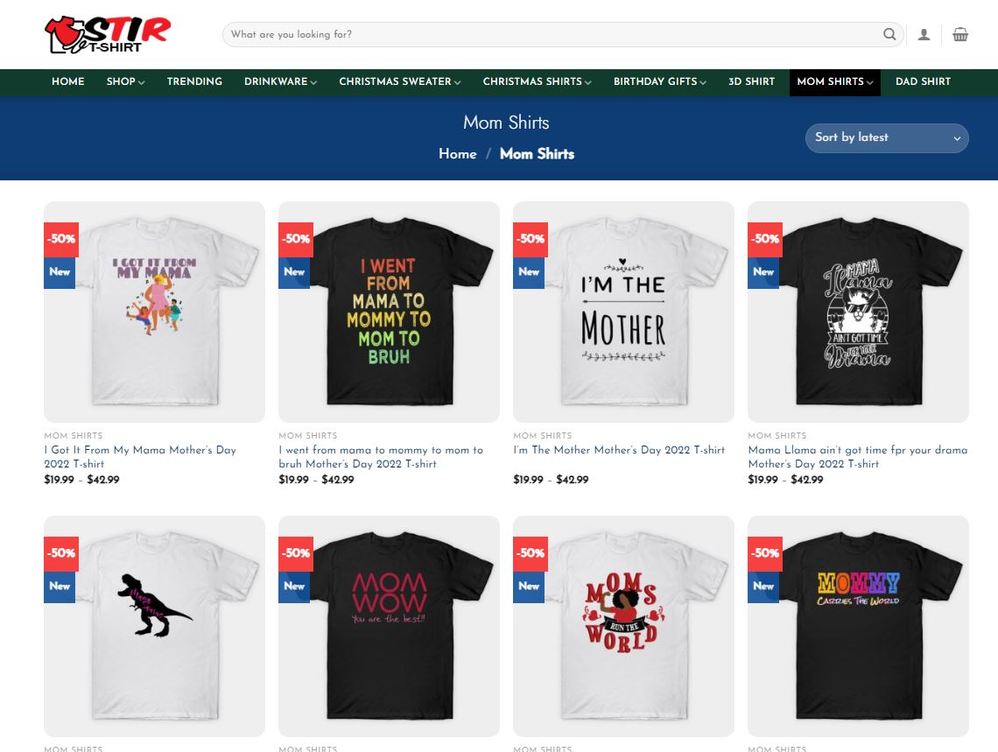The image depicts a website for a t-shirt company named "STIR T-Shirt." The logo features the word "STIR" in all capital letters, with alternating colors: the S and I in black, and the T and R in red. To the left of the logo is an illustration of a red t-shirt. Just below the logo, there's a search bar with the placeholder text "What are you looking for?".

A black navigation bar beneath the search bar contains white, all-cap letters for the categories: HOME, SHOP, TRENDING, DRINK WEAR, CHRISTMAS SWEATER, CHRISTMAS SHIRTS, BIRTHDAY GIFTS, 3D SHIRT, MOM SHIRTS, and DAD SHIRTS. The "MOM SHIRTS" category is currently selected. Below this section, a larger blue bar prominently displays the text "MOM SHIRTS," with a breadcrumb trail below reading "Home / Mom Shirts." On the right side of this blue bar, there's another search functionality labeled "Sort by Latest."

The main content area shows a grid of eight t-shirts, organized in two rows of four. Each t-shirt is detailed as follows:

1. **Top Left**: A white t-shirt with the text "I got it from my mama" featuring a mom in the center with two kids on either side, marked as "50% Off New." It is titled "I got it from my mama, Mother's Day 2022 T-shirt" and priced between $19.99 and $42.99.
   
2. **Top Second**: A black t-shirt with rainbow-colored lettering that transitions from red to green, stating "I went from mama to mommy to mom to bra," priced similarly at $19.99 to $42.99.

3. **Top Third**: A white t-shirt with black lettering that says "I'm the mother," available for $19.99 to $42.99.

4. **Top Right**: A black t-shirt featuring a white logo with the text "Mama Llama ain't got time for your drama" accompanied by an image of a llama, also priced between $19.99 and $42.99.

5. **Bottom Left**: A white t-shirt with an illustration of a T-Rex facing left with its mouth open, without any additional text or pricing details provided.

6. **Bottom Second**: A black t-shirt with red text "Mom WOW" followed by the phrase "You are the best," no additional pricing or description provided.

7. **Bottom Third**: A white t-shirt with the text "Moms Around the World" featuring a black mom at the center and red text, no pricing provided.

8. **Bottom Right**: A black t-shirt with multi-colored letters spelling "Mommy carries the world," with the text "Mommy" in yellow, orange, red, blue, and purple, without further pricing details.

Overall, the website offers a visually appealing and well-organized layout, specifically highlighting t-shirts for mothers with creative and diverse designs, suitable for occasions such as Mother’s Day 2022.